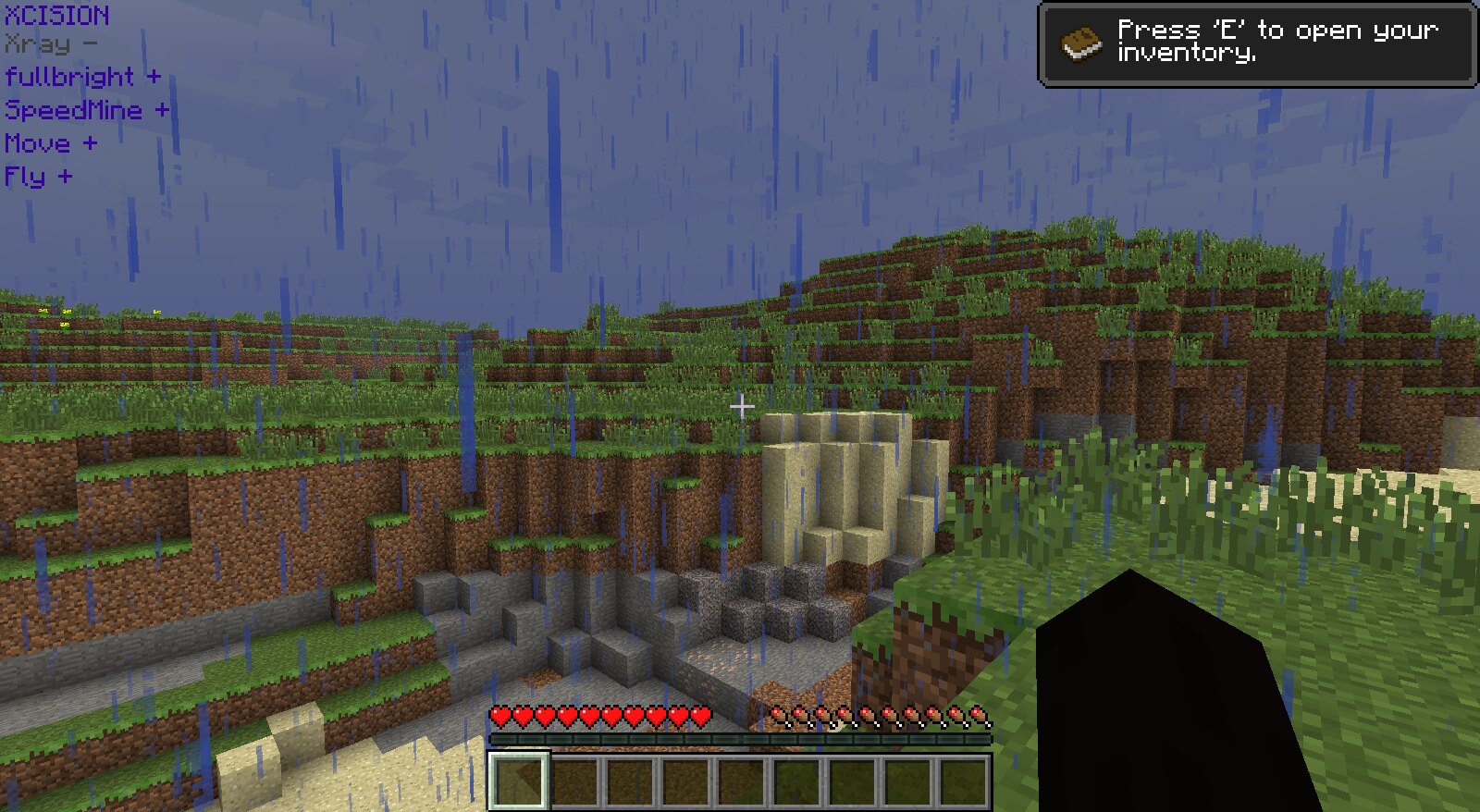This is a detailed screenshot from the game Minecraft, captured in a first-person perspective. The scene features a rugged, mountainous region with a mix of gray and sandy bricks, dirt, and grass textures topping the cliffs. In the foreground, the player holds a default tool, indicative of a first-person view. The sky above is pixelated, blue with clouds, and it's raining, noted by the falling blue pixels. There are ten hearts displayed, signaling full health, and the inventory bar along the bottom shows empty slots. Text overlays in the image provide various instructions and indicators: "Press E to open your inventory" appears in a small box in the top right corner next to a book symbol, while the top left corner features a series of commands such as "excision," "x-ray minus," "full bright plus," "speed bind plus," "move plus," and "fly plus." The view may resemble an auditorium-like area with tiered plants, reflecting the versatile building and environmental dynamics of Minecraft.